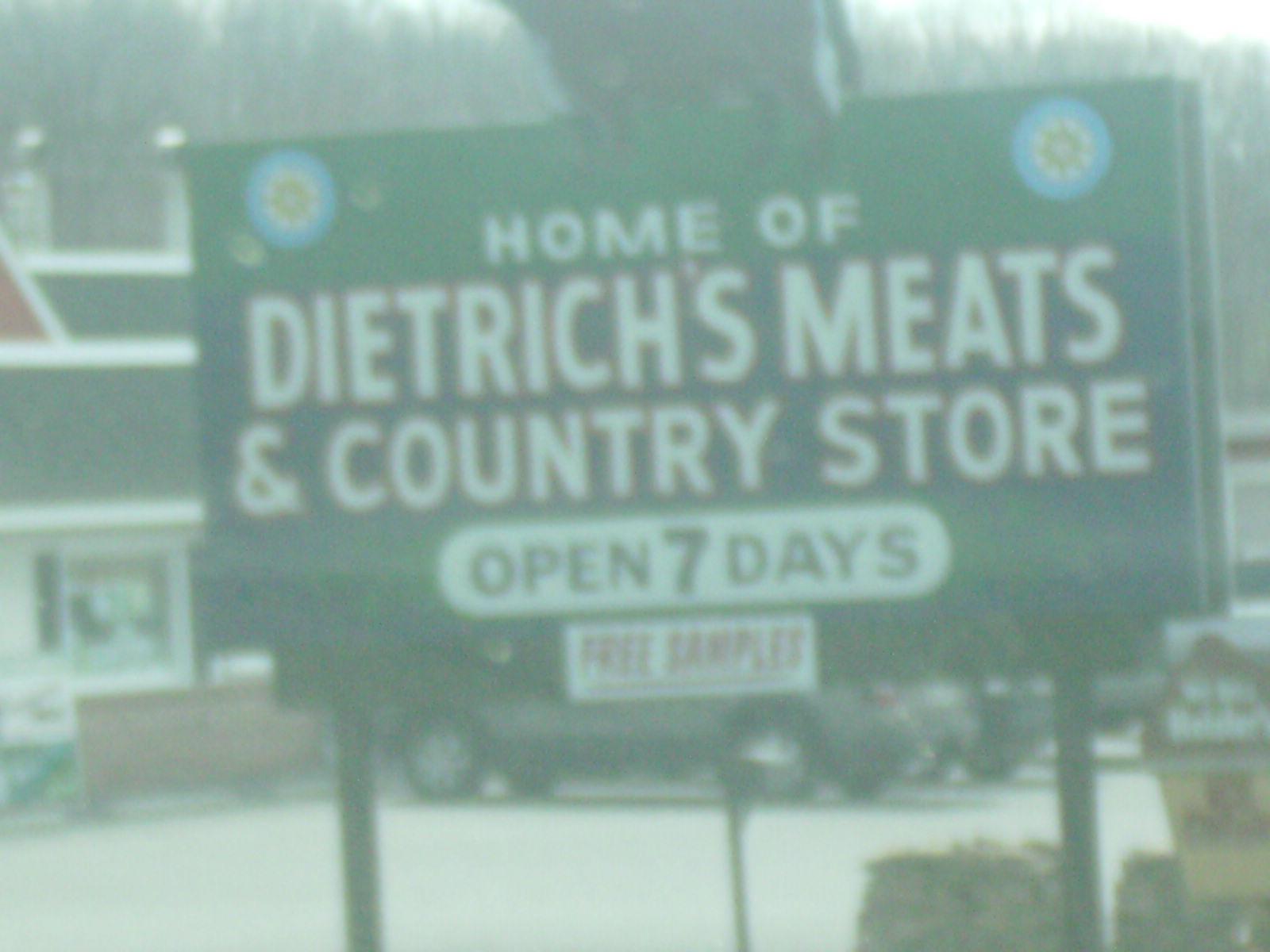The photograph captures a somewhat faded and hazy image that is slightly wider than it is tall, contributing to a washed-out effect that might be due to fog or another environmental factor. Dominating the foreground is a low-to-the-ground dark green sign with white and red outlined text, stating "Home of Dietrich's Meats and Country Store." The text is center-aligned across five lines, and additional details mention the store is "open seven days" with "free samples." The phrase "open seven days" is highlighted within a white oval. Notably, the top corners of the sign feature blue circles with yellow flowers inside.

Flanking the sign are two black poles, with a row of cars parked diagonally at around 9:30 behind it. In the background stands the country store, characterized by its white upper half, a black roof outlined in white, and possibly a red-brick lower half or front of the building. The roof also has a distinct red segment. The store has windows, one of which contains an unreadable sign from this distance. Additional background elements include bare trees, what appears to be some bales of hay, and possibly a smaller sign advertising ice cream or milkshakes located in the bottom right corner of the frame. Overall, the photograph combines elements of rural charm with the welcoming promise of Dietrich's Meats and Country Store.